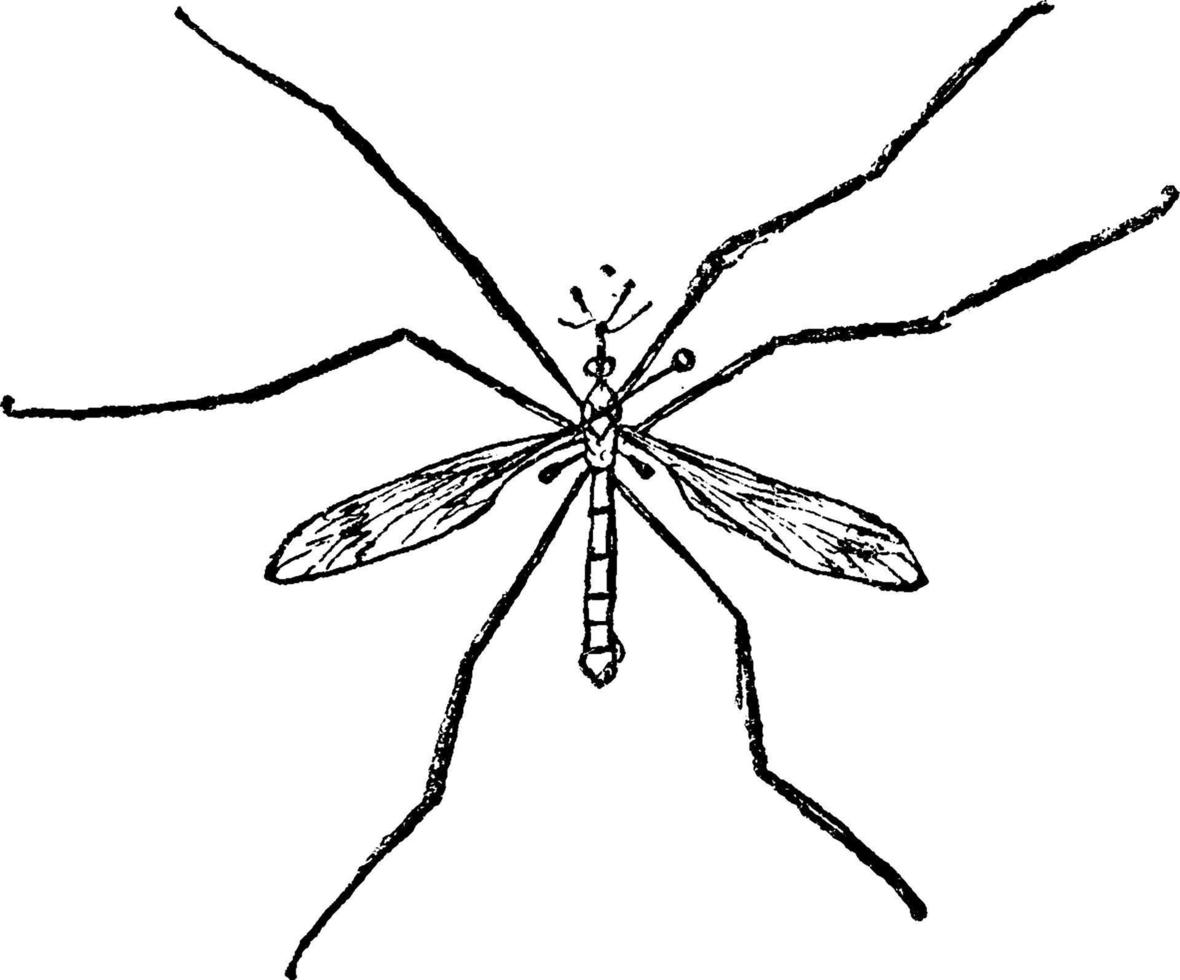This hand-drawn illustration, rendered in a simple black-and-white sketchy style, features a detailed but minimalistic depiction of an insect, likely a mosquito given its prominent features. At the center of the drawing, the mosquito has a long, slender body segmented into different compartments, topped with a head characterized by two large eyes and multiple short antennae. It sports two translucent wings with detailed webbing emerging from the middle of its thorax. The insect's six legs, articulated at the joints, extend towards the edges of the canvas, giving it a lifelike pose. While the wings are slightly asymmetrical, they remain attached centrally. The illustration uses a rough texture, possibly achieved with crayon, charcoal, or pencil, enhancing the simple yet expressive nature of the image.